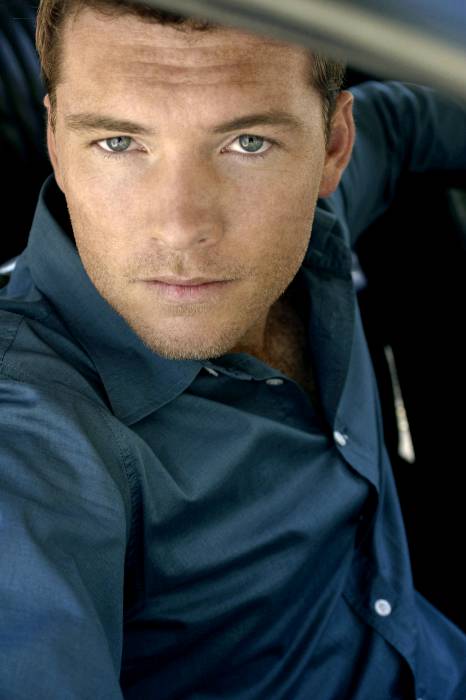The image is a close-up of a young man with short brown hair and a light stubble beard, looking directly into the camera with piercing light blue eyes. His face is covered in freckles, notably on his forehead. He is wearing a greenish-blue or navy collared button-down shirt with white buttons, slightly open at the top. The background is dark, with hints of light and silver suggesting an opening behind him. There is a curved bar or handle at the top part of the frame, possibly part of a car's doorframe, giving the impression he might be inside a vehicle. His expression is neutral, and he appears to be leaning into the car, possibly closing the door.